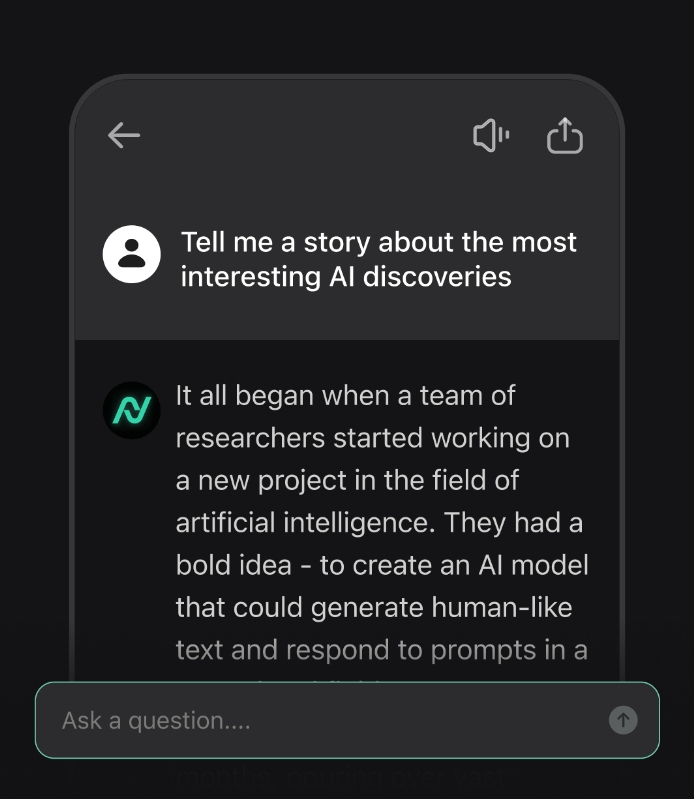A user is interacting with an AI chatbot, likely ChatGPT, within an application featuring a sleek, dark grey interface. The chat window itself is a slightly lighter grey, topped with a very pale grey arrow pointing to the left, and includes a sound icon and an upload arrow (an arrow pointing upwards from a rectangular shape with rounded edges) on the far right. The user’s profile picture is a simple white circle with a black human icon inside. 

The user has asked, "Tell me a story about the most interesting AI discoveries." The chatbot's response begins with a black circle featuring a green icon with two squiggly lines and reads, "It all began when a team of researchers started working on a new project in the field of artificial intelligence. They had a bold idea to create an AI model that could generate human-like text and respond to prompts in a..." but the message is cut off. 

Below this exchange, there’s a text input box where users can type their queries, alongside an upward-pointing arrow icon used to submit the text.